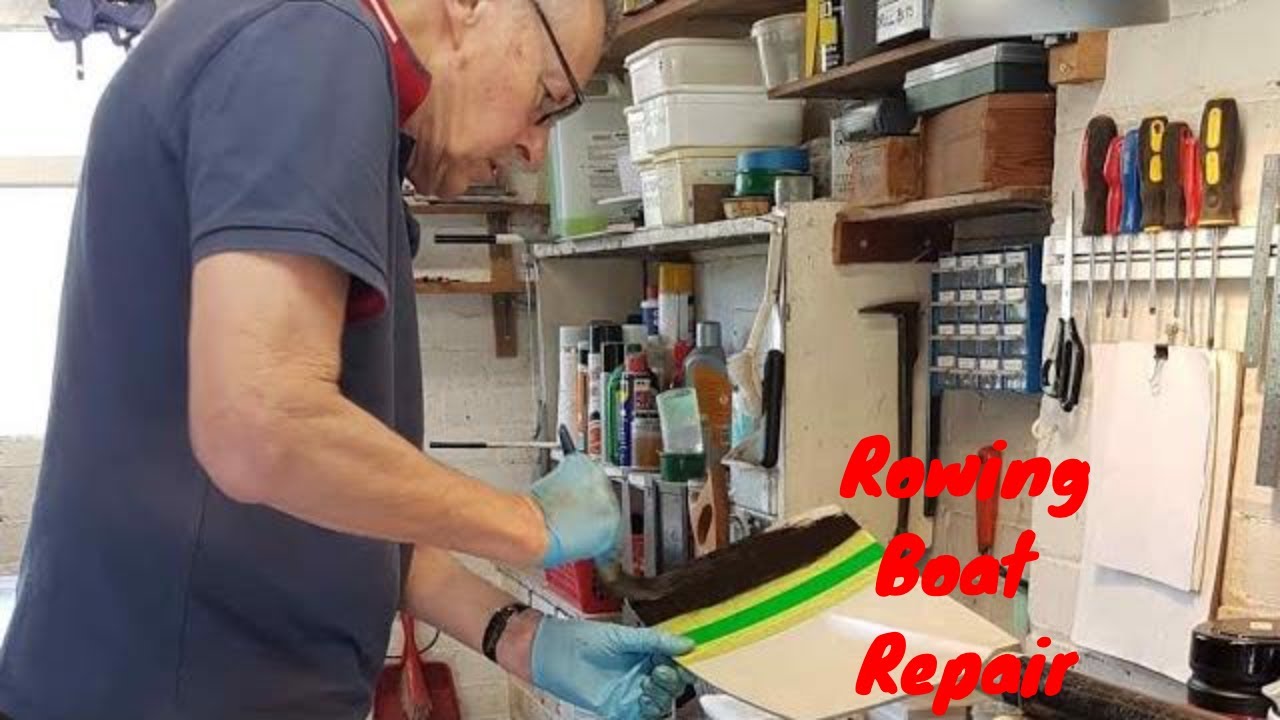The detailed photograph captures an elderly, bald, white man, approximately 75 years old, deeply engrossed in his work within a cluttered yet organized garage workshop. He is wearing glasses, a blue shirt, and blue latex gloves, and is positioned centrally in the image, focusing intently on an object he is holding. The text "Rowing Boat Repair" in bold red letters is visible at the bottom right corner, indicating his specialized craft—repairing rowing boats. The man appears to be applying either paint or glue to a primarily white object adorned with green, yellow, and brown stripes. His workspace against the wall is lined with various colored screwdrivers, systematically arranged from big to small, alongside multiple boxes of materials and tools neatly stacked on wooden shelves, reflecting the essence of his diligent and organized work environment.